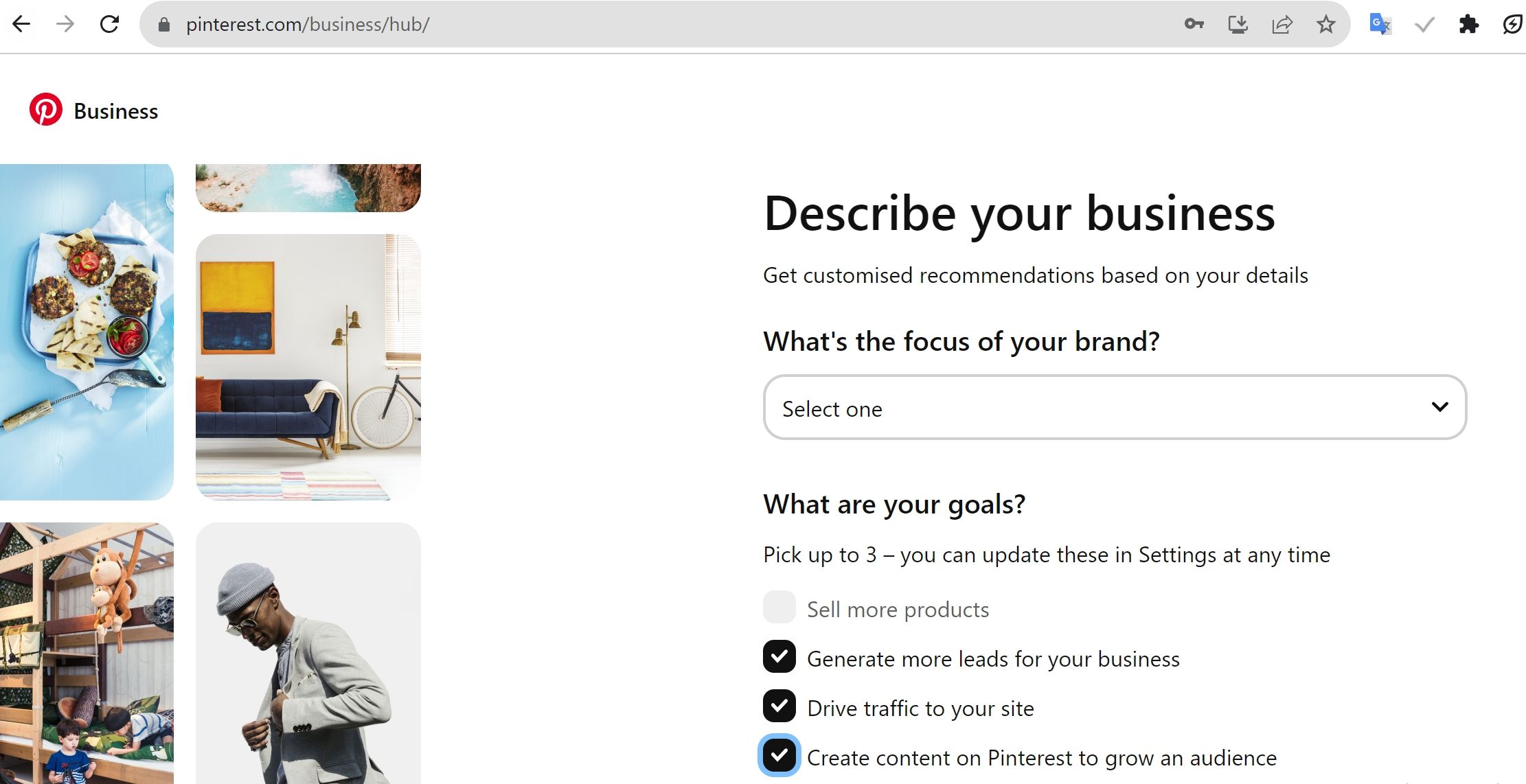**Detailed Caption:**

The image displays a web browser window open to the URL "pinterest.com/business/hub/." In the browser's address bar at the top, navigation icons are visible, including arrows pointing left and right for backward and forward navigation, respectively, and a circular arrow for reloading the page. On the right side of the address bar, there are additional icons: a key, a download symbol, a symbol with an arrow pointing to the right, a star, the letter "G," a checkmark, a jigsaw puzzle piece, and an unrecognized symbol.

Beneath the address bar, against a white background in the upper left corner, the red Pinterest logo is prominently displayed, followed by the word "Business." Below this heading, there are small, square photographs: the first is of food on a plate, the second is a partially visible image of a waterfall, the third shows a living room featuring a couch and a bicycle, the fourth is of a man in a suit wearing a knit cap, and the fifth depicts two young boys on a bunk bed.

On the right side of the page, there is a heading titled "Describe your business," accompanied by an icon. Below this heading, the text reads, "Get customized recommendations based on your details. What's the focus of your brand?" This is followed by a search box resembling an oval rectangle with the placeholder text "Select one" and a drop-down arrow for options. Further down, the text inquires about the user's goals with the line, "Pick up to three. You can update these in settings at any time." Four goal options are listed with corresponding checkboxes: 

1. "Sell more products" (unchecked)
2. "Generate more leads for your business" (checked)
3. "Drive traffic to your site" (checked)
4. "Create content on Pinterest to grow an audience" (checked)